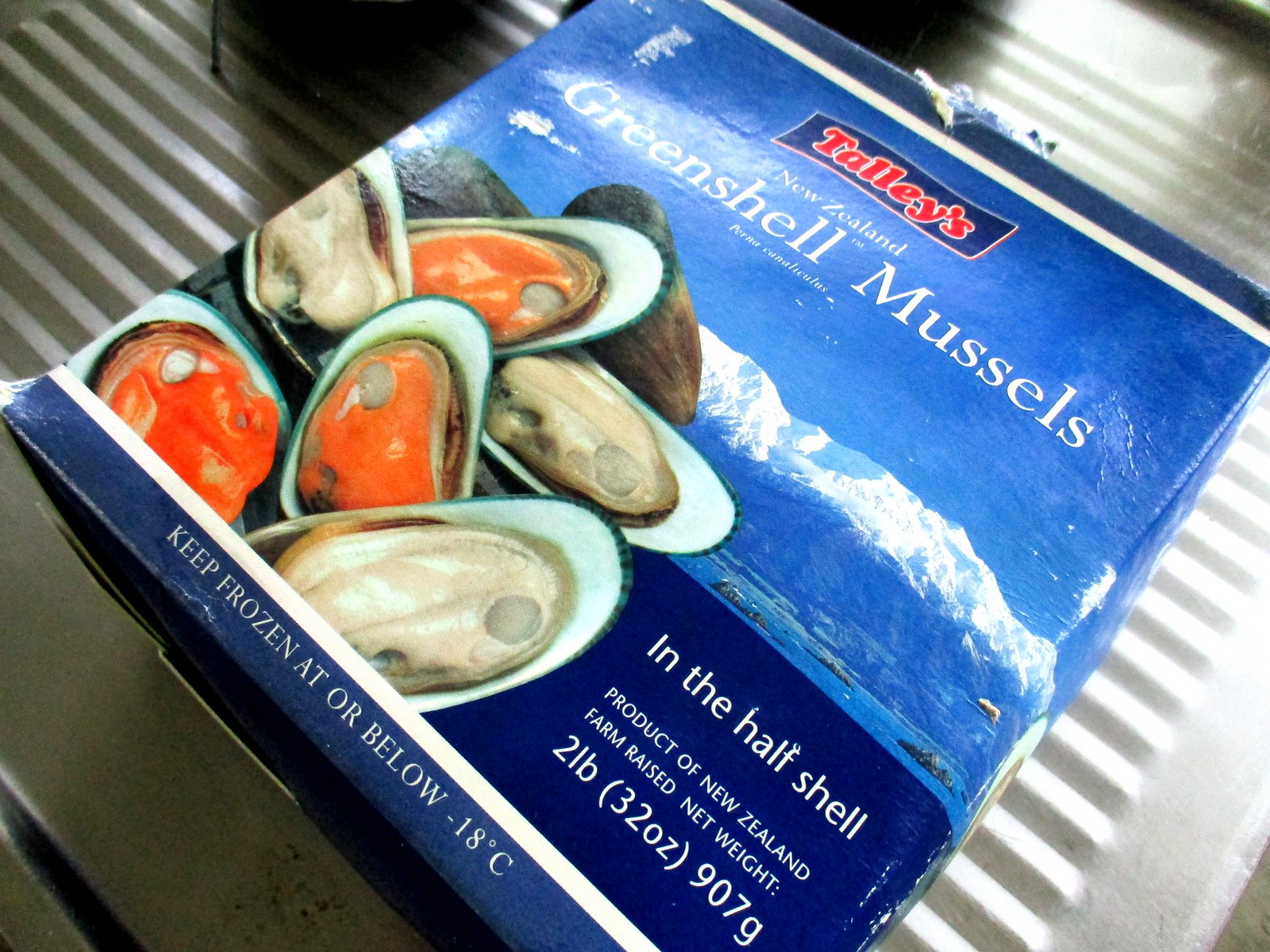The photograph is a rectangular image showcasing a package of frozen mussels against a silver, grooved, washboard-like countertop, possibly part of a cooktop or grill with black dials at the top. The blue box prominently displays the brand name "Tally's" in red text on a white line across the top. Below the brand name, in white text on a blue background, the package reads "New Zealand Green Shell Mussels" along with "Perna canaliculus" underneath.

The packaging features an idyllic mountain scene with snow-capped peaks, brown slopes, blue water, and rocks, serving as a backdrop for the image of mussels on the half shell. These mussels vary in color from whitish-gray to pinkish-orange, surrounded by white edges and housed in brown shells.

Additional text on the package reads "In the Half Shell," "Product of New Zealand," and "Farm-Raised." The net weight is provided as "2 pounds (32 ounces) or 907 grams." At the bottom, a blue bar with white text instructs, "Keep Frozen at or Below -18°C" ensuring proper storage instructions. The package itself is slightly tilted to the right, adding a dynamic element to the image.